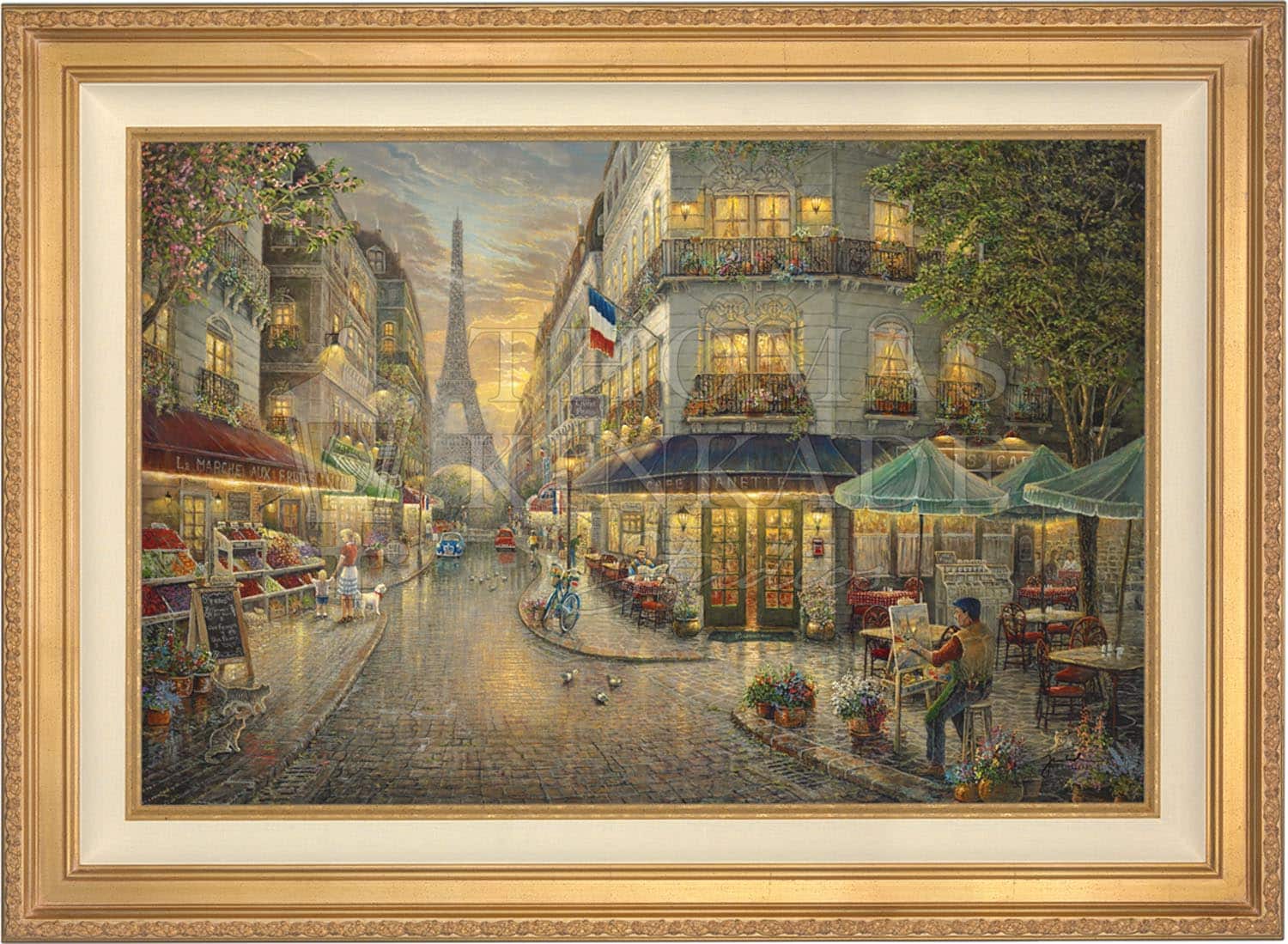This framed painting, set in a horizontal orientation, features an ornate, gold-colored frame adorned with an intricate, decorative pattern. Encased within the frame, a matte white border surrounds the inner gold trim that leads directly to the painting itself. The scene within the painting depicts a charming Parisian street, with the iconic Eiffel Tower visible in the background, firmly establishing the setting as Paris. Flanking the cobblestone street are various shops, and a notable detail is the French flag with its blue, white, and red stripes displayed in the upper right corner. A man is positioned at the lower right of the painting, seated at a stool beneath a parasol, busily painting the very same scene we observe, creating a painting within a painting. This scene is rich in warm hues, with lights illuminating the buildings, and there is a subtle watermark over the image. The overall ambiance is one of quaint, bustling charm typical of a Parisian boardwalk area.